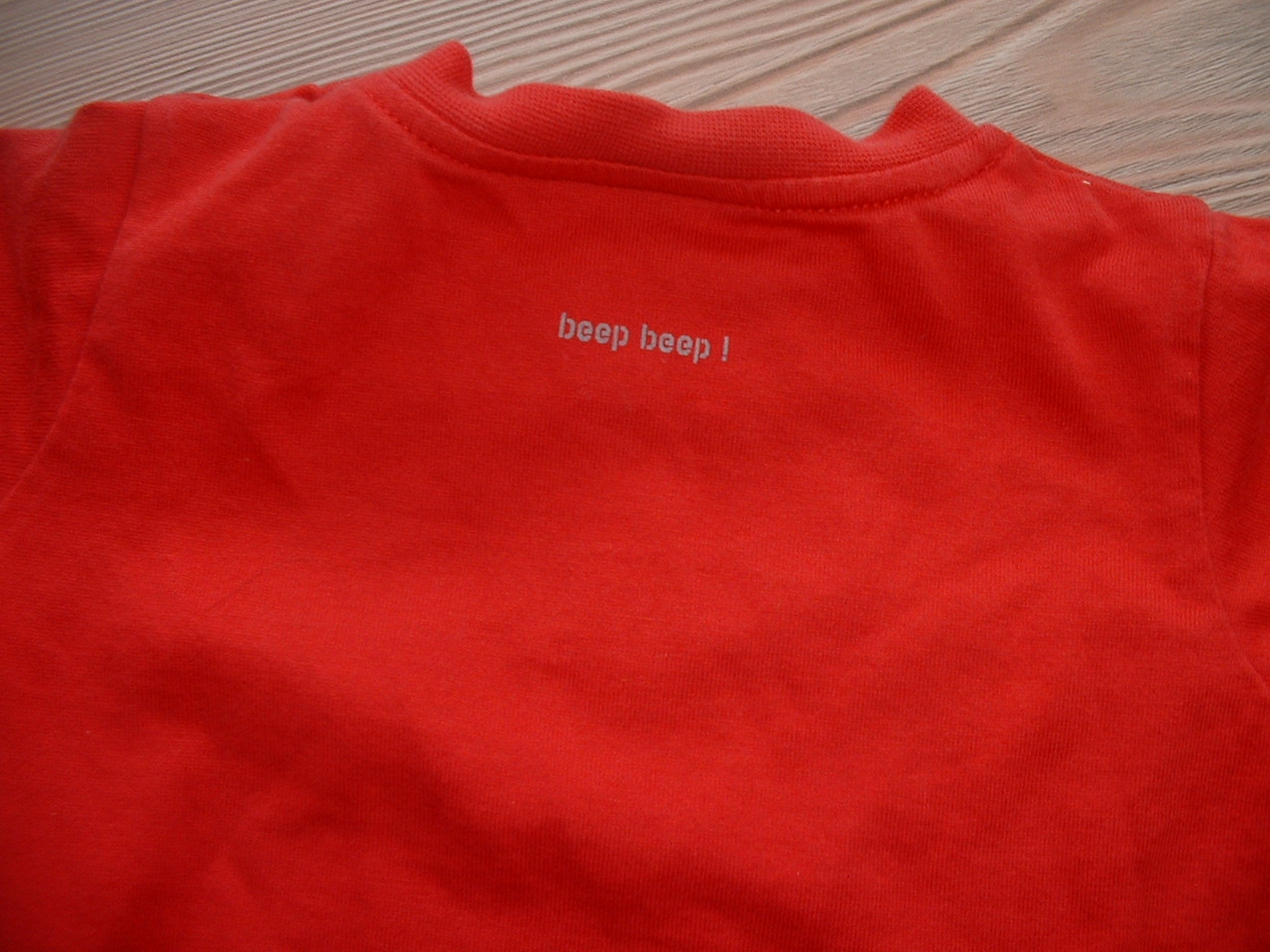A vibrant tomato-red cotton T-shirt is displayed with its back facing up. Positioned approximately an inch below the collar, the phrase "Beep Beep!" is printed in bold letters. The neckline of the shirt appears reinforced, suggesting durability, and the sleeves are short, typical of a standard T-shirt design. The T-shirt is laid out flat on a light-colored, natural wood table, showcasing the wood's organic grain patterns and marks, highlighting its unstained, authentic finish.